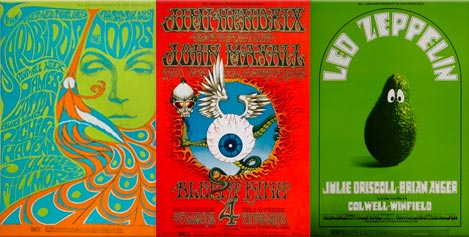The image depicts a set of three vintage psychedelic music posters. 

The left poster features a bright blue background with neon green, psychedelic text that's difficult to read but includes the names Yardbirds, Doors, and James Cotton. A stylized woman's face with arched eyebrows, the same color as the green text, is on the right side. The center of this poster showcases a stylized peacock design with orange, blue, and white feathers, adorned with green circles. 

The central poster highlights the names Jimi Hendrix and John Mayall with funky lettering at the top. Dominating the center is a vividly painted veiny eyeball with a blue iris, sprouting white and brown wings. It has tentacles: one lifting a flaming-eyed skull, another holding open a fiery hole the eye is crawling through, and a third coiling around. At the bottom, the number four appears in drippy text, accompanied by blocks of illegible small text on either side. 

The right poster has a warm green background with a black, curved door-shaped outline at the top. Following this curve, the text reads Led Zeppelin. The central image is a dark green avocado with googly eyes, resembling a face. Below, in white text, are the names Julie Driscoll, Brian Auger, and Colwell Winfield, followed by two lines of tiny black, illegible text.